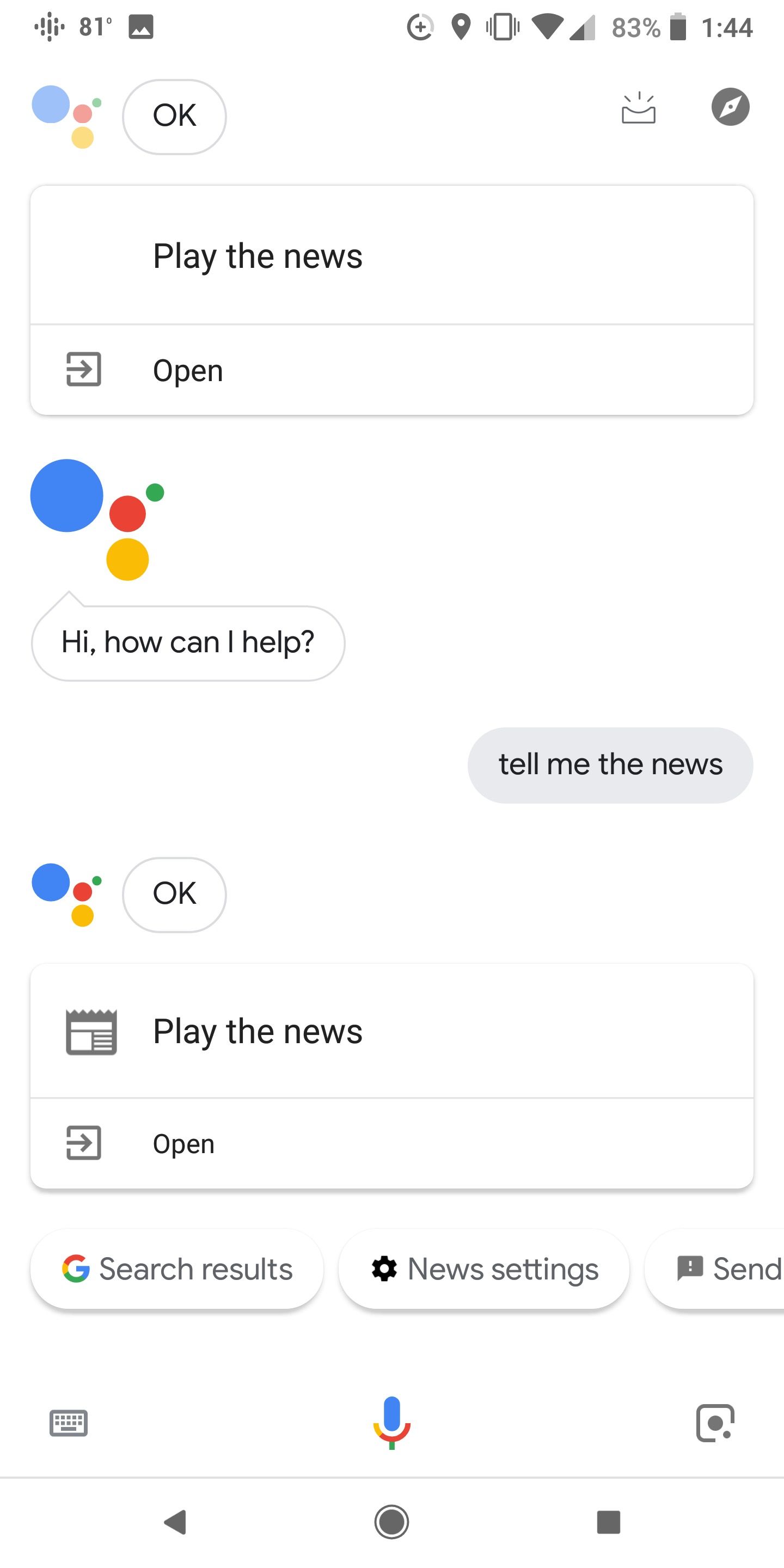The image depicts a screenshot of an Android device in portrait mode. At the top of the screen, status icons are visible, showing the time, battery level, Wi-Fi signal, and temperature, characteristic of an Android phone interface. 

At the bottom, navigation icons are present: a triangle, a filled circle, a bordered circle with some spacing around it, and a square. 

The main content of the screenshot appears to be a chat or interaction with a bot. The top portion of the chat interface displays a series of dots: a larger blue dot, a medium-sized orange dot, a red dot slightly smaller than the orange, and a very small green dot. Just above these dots, the word "Okay" is displayed alongside options to "Play the news" or "Open."

Beneath this, a wide, horizontally oriented, rounded rectangle distorts slightly upwards at the corners. Inside this rectangle, the bot or assistant greets with "Hi, how can I help?"

It seems the user may have prompted "Tell me the news," as indicated by the subsequent content. Below the assistant's greeting, the familiar dot icons appear again, followed by a smaller rounded rectangle containing the button label "OK" in capital letters.

Further down, there are two rows within boxes. The first row features an icon followed by the text "Play the news." The second row also contains an icon and the text "Open."

At the bottom of this interface are three distinct buttons. The first button displays the colorful "G" logo of Google with an accompanying label "Search results." The second button shows a gear icon labeled "News settings." The third button has a chat bubble icon with an exclamation point inside, with the word "Send" truncated.

Finally, three additional icons are positioned at the absolute bottom of the screen: a keyboard icon on the left, a multicolored microphone icon in the center typical of Google’s voice input, and to the right, a square with rounded corners but a dot where the lower right corner should be.